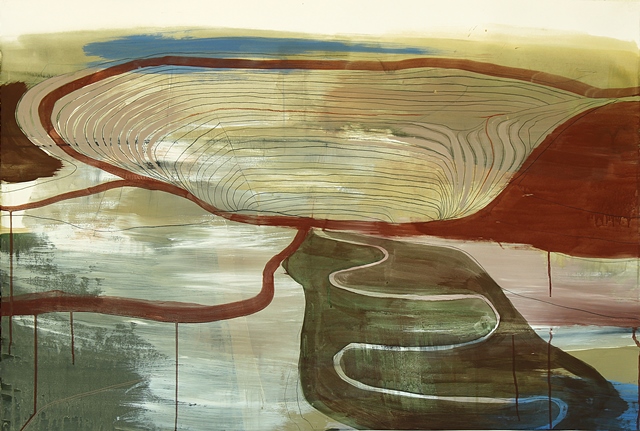The artwork is an abstract painting with a horizontal orientation, characterized by a variety of swirling and flowing effects that lend it a water-like feel, possibly created using watercolors. Dominant colors include red, green, and blue, accompanied by touches of tan, white, and black. The image features a prominent red circular shape situated to the right of the center, from which several thinner red lines and streaks appear to drip downward. This red circle encloses irregular shapes filled with mixtures of black, white, and gray, and is bordered on either side by winding, river-like white lines that snake through the composition, creating a mirroring effect between the top and bottom halves of the painting.

The top of the image includes a thin strip of light colors, ranging from white to light gray, under which patches of blue dominate the left side and tan stretches across the middle. Below this, the painting transitions into the central red area, outlined in bold, where additional red streaks and smudges appear to drip toward the bottom. These red strokes define irregular shapes containing light grays and greens.

At the bottom left, there's a notable green section, contrasting with an area of brownish and dark gray tones that surround the central winding white line. Accentuating this natural, reflective quality, the bottom right corner of the painting features subtle pops of purple and blue, accompanied by areas of smudged white, tan, and reddish tones. Through a blend of colors and flowing lines, the painting evokes a sense of a puddle reflecting a complex, colorful sky.